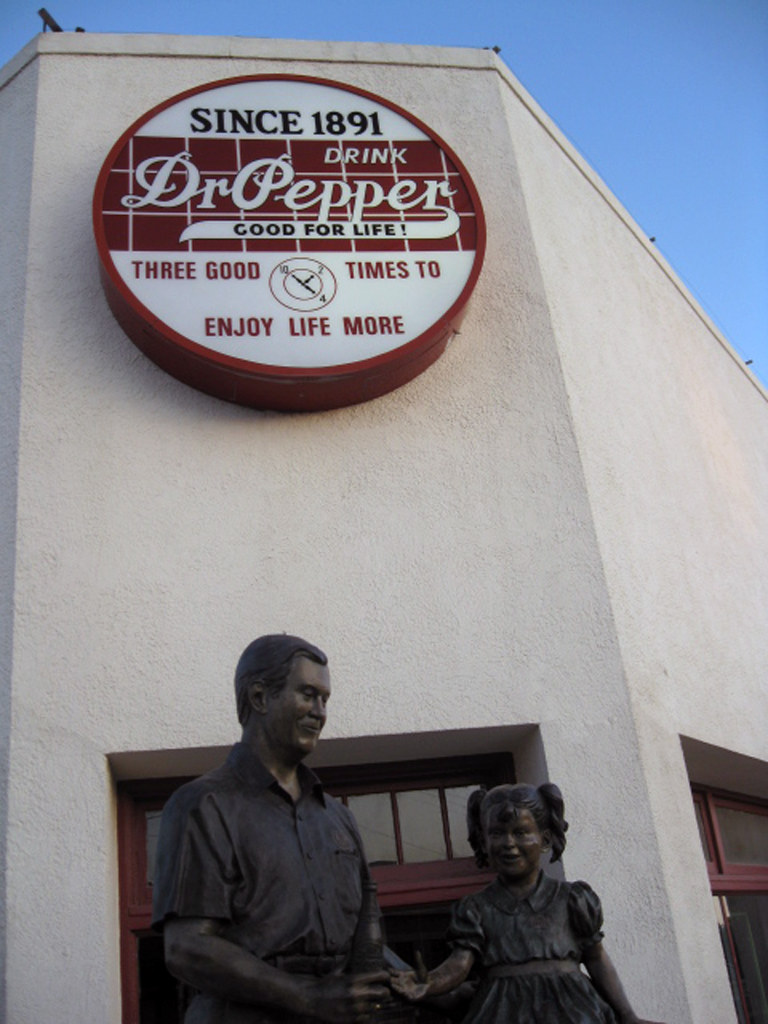The photograph captures a bronze statue of a man and a girl, positioned in front of a white, rectangular building adorned with wooden-framed doors. The statue depicts a smiling man, visible from the waist up in a button-up shirt, handing a bottle to a girl with her hair pulled back into pigtails, wearing a short-sleeved dress. Behind them, a prominent large round sign in red and white reads, "Since 1891, Drink Dr. Pepper, Good for Life," accompanied by a clock with hands positioned at 10, 2, and 4, and the phrase "Three good times to enjoy life more." The scene is set against a clear blue sky, making the statue and the Dr. Pepper sign striking focal points of the image, hinting at a long-standing tradition embraced by the iconic brand.